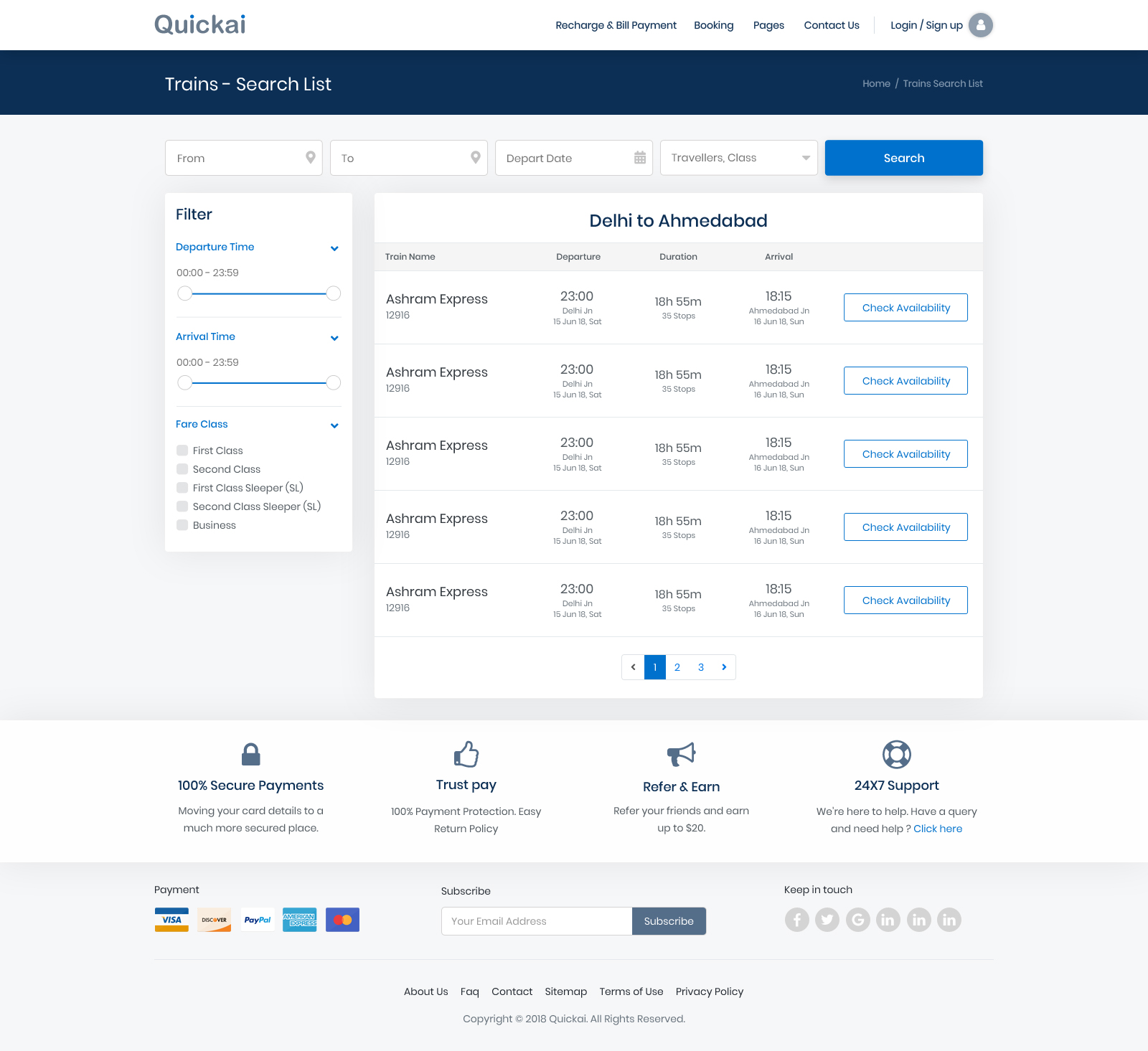This image depicts a webpage from a platform called "QUICAI," spelled Q-U-I-C-K-A-I, with the name prominently displayed in gray text at the top. Beneath the platform's name, there is a dark navy navigation bar featuring options such as "Trains," "Search List," "Recharge and Bill Payment," "Booking Pages," "Contact Us," and a circular gray icon for "Login/Sign Up." 

The primary section of the page is dedicated to booking trips, starting with input fields for "From Date," "To Date," "Departure Date," and "Traveler's Class." These fields are set against a light gray background, with white input boxes for typing the required information. The "Traveler's Class" has a dropdown menu to select different classes, while the other fields require direct input. A prominent blue "Search" button is positioned to the right of these input boxes.

Below the search section, there is a white filter box which allows users to customize their search by departure times and fare classes through checkboxes. Displayed prominently is a sample route from Delhi to Ahmedabad, showcasing various train options and their availabilities. Each train option includes specifics and an availability check button, which is white and outlined in blue, with the text "Check Availability" in blue as well.

The footer of the webpage highlights key service features like "100% Secure Payments," "Trust Pay," "Refer and Earn," and "24/7 Support," along with an array of accepted credit card logos, reassuring users of secure and versatile payment options.